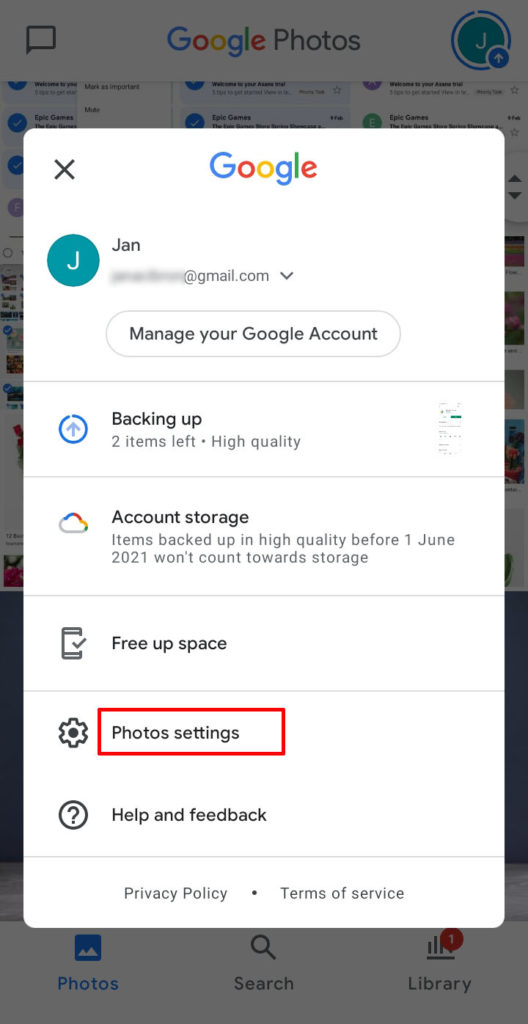This detailed caption describes an image featuring a screenshot of a small settings or pop-up window with various account and backup details.

---

The screenshot displays a small settings or pop-up window, centrally focused, with the header text starting with "Jan." Below the header, a portion of a blurred-out email address is partially visible, ending with "@gmail.com." A status update reads, "Backing up, two items left," followed by "high quality." The next section provides information on account storage, stating that "items backed up in high quality before June 1st, 2021 won't count towards storage." 

There are actionable buttons labeled "Free up space," "Photos," and "Settings," with the latter two encapsulated in a red box, indicating their prominence or a user's selection. The final line of text at the bottom of the window offers "Help and feedback."

---

This descriptive caption offers a clear, structured overview of the screenshot's key elements and layout.